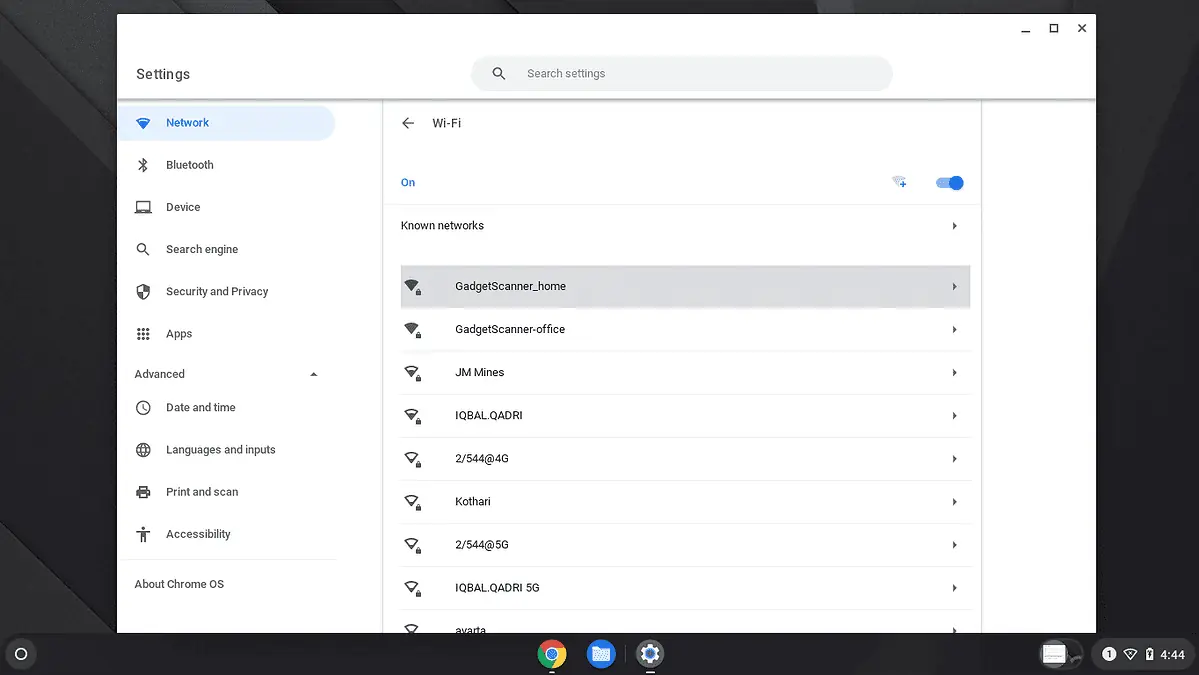A computer screen displays a minimized window, surrounded by a black background. The dock at the bottom of the screen features various icons, including Google Chrome, Microsoft Word, a file folder, and an unrecognized symbol. The central part of the screen shows a white document window that can be minimized, expanded to full screen, or closed. This window appears to be settings-related, featuring a search bar in the middle.

On the left side of the document, there's a vertical menu listing several options:
- Network (highlighted in blue)
- Bluetooth
- Device
- Search Engine
- Security and Privacy
- Apps
- Advanced

Under "Advanced," additional options include:
- Date and Time
- Language and Inputs
- Print and Scan
- Accessibility
- About Chrome OS

In the middle of the screen, within the Network settings, Wi-Fi is turned on and connected to a network labeled "Gadget Scanner Home," which is grayed out, indicating the current connection. Other networks are listed, including "Gadget Scanner Office," which is not selected. The detailed layout and options indicate that the user is actively managing or reviewing network settings and other system configurations.